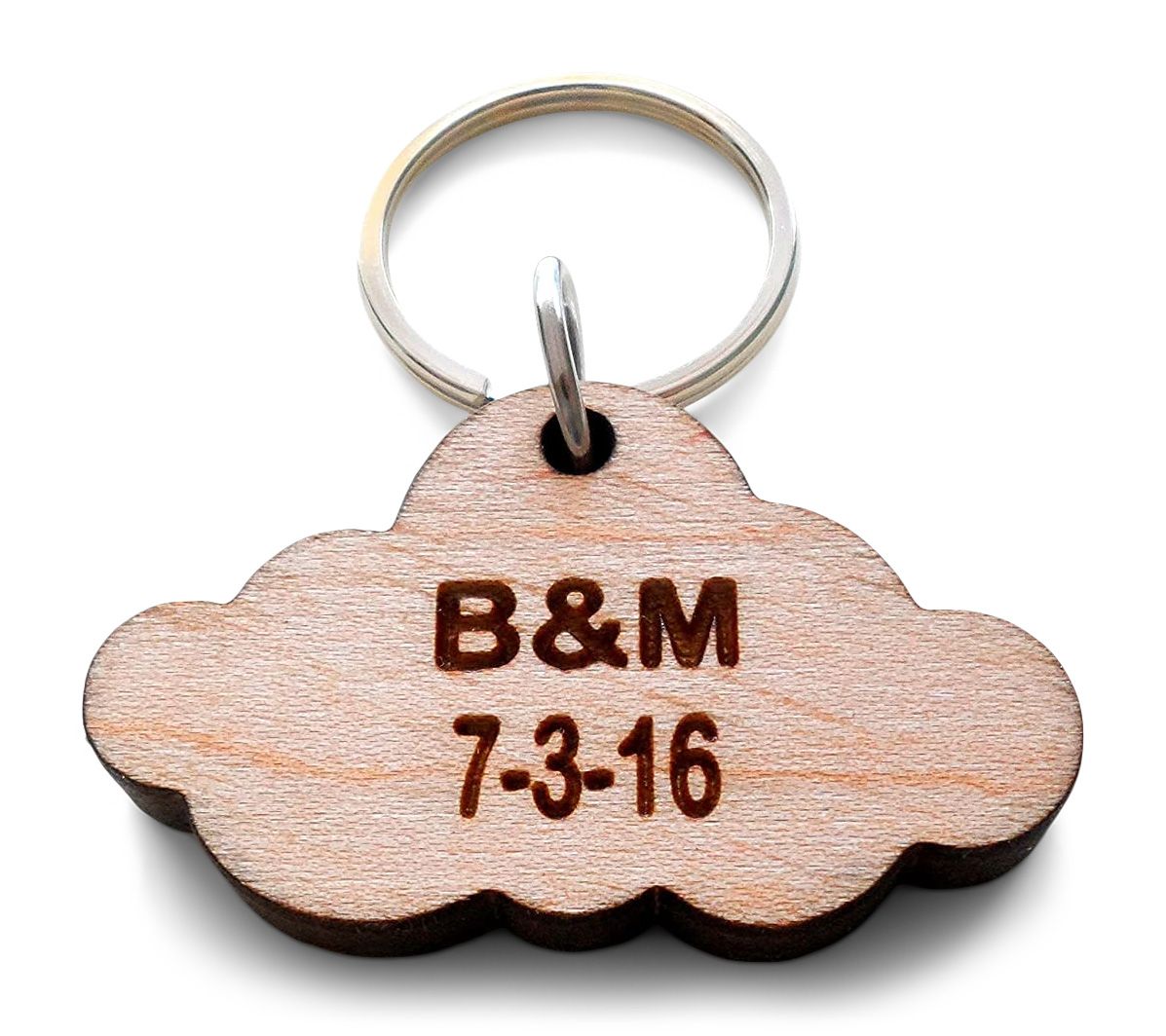The image features a close-up of a keychain against a completely white background. The keychain consists of a silver, chrome-colored ring at the top, connected to a wooden cutout via a silver link. The wooden cutout is meticulously shaped like a cloud and exhibits clear, sanded wood grain. Engraved in dark brown on the wood are the letters "B" and "M" with an ampersand sign in between, followed by the date "7-3-16" beneath them. The edges of the cloud-shaped wooden piece are distinctly dark brown, suggesting they were burned to create a weathered yet intentionally crafted appearance. The overall presentation of the image implies it could be a product photo, possibly for a website selling personalized items such as animal tags, emphasizing the fine details and craftsmanship of the keychain.